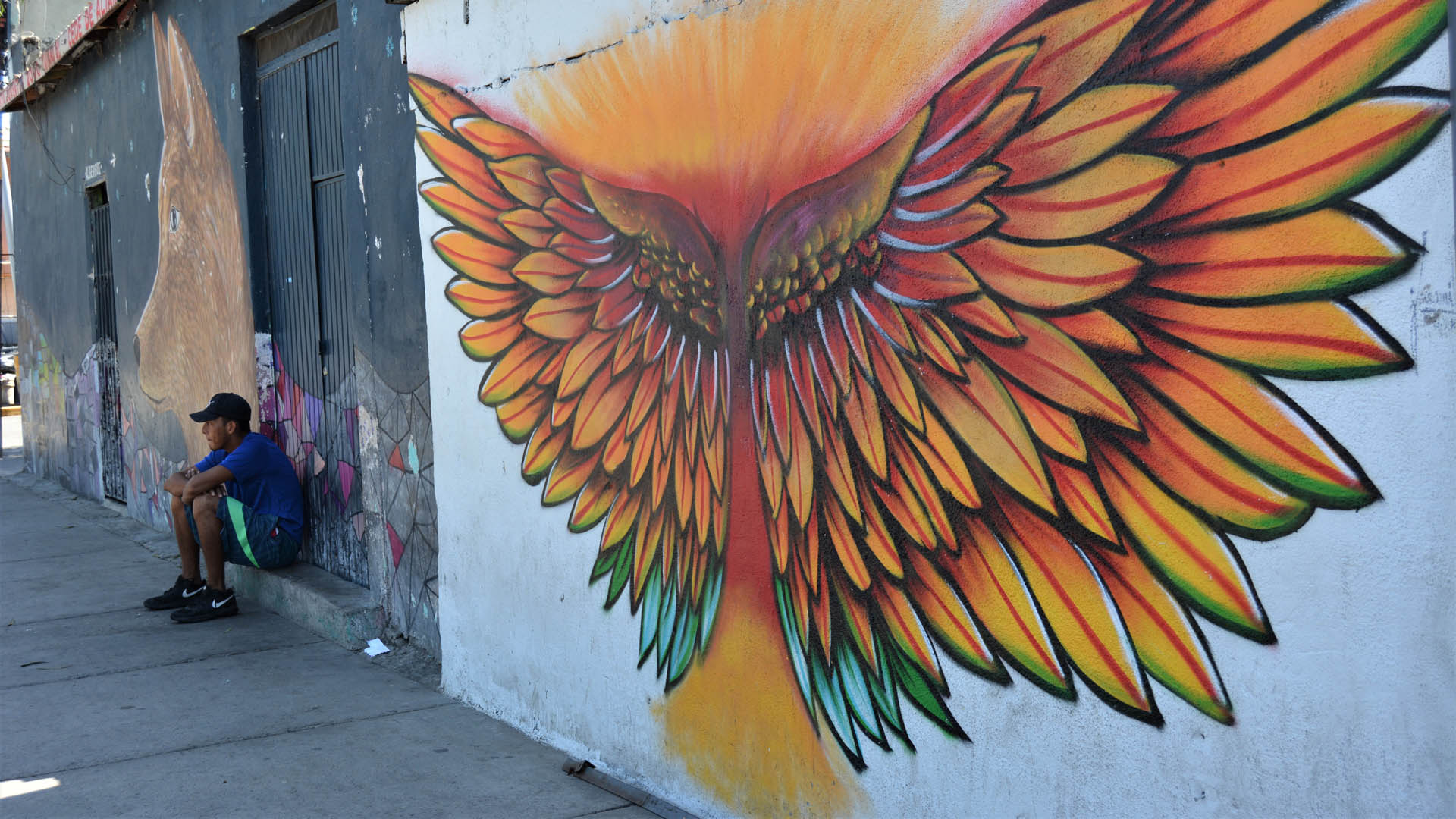The photograph captures an outdoor urban scene featuring a man resting on a concrete pillar beside a black building adorned with vibrant street art. The man, wearing a black hat and black tennis shoes, looks off to the left as he sits on a step. Behind him, a mural on a black wall depicts the face of a brown wolf or coyote. To the right, closer to the camera, stands a white wall embellished with colorful wings painted in orange, green, and red, resembling sunflowers. These wings, created with spray paint, emanate a radiant combination of colors. The background of the mural features vivid reds and oranges, with a sidewalk visible on the left side. The scene appears to be set early in the day, illuminated by sunlight enhancing the brilliant hues of the graffiti art.